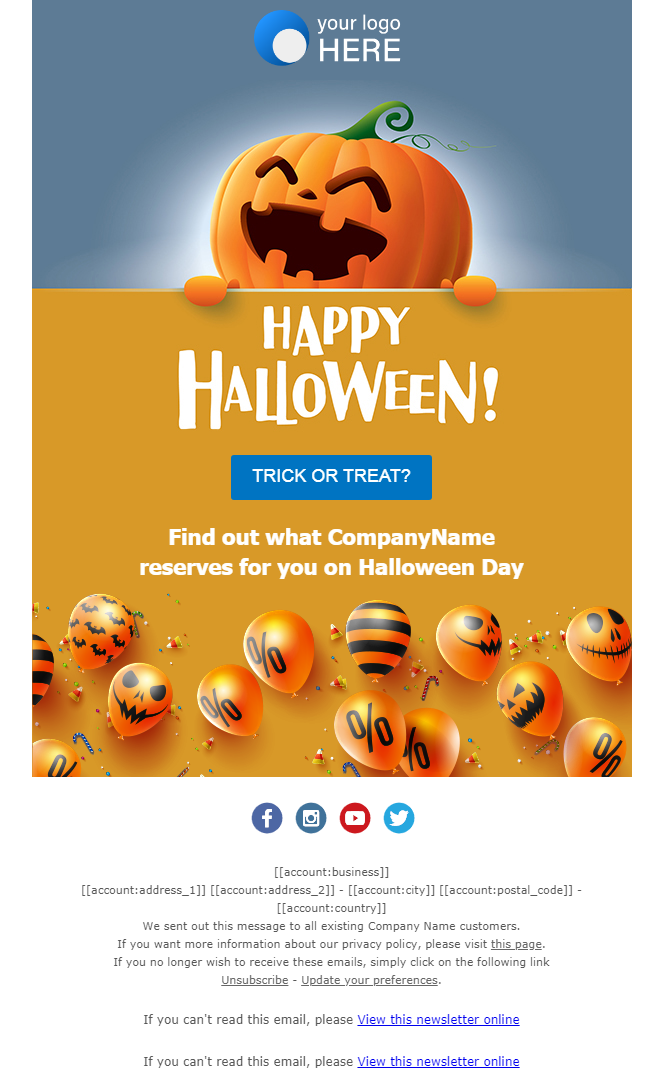This detailed summary image captures the essence of a festive Halloween newsletter. At the top, there is a placeholder for the company logo with a cheerful "Happy Halloween! Trick or Treat" greeting. The newsletter teases readers with an intriguing message: "Find out what [Company Name] reserves for you on Halloween Day," suggesting exclusive offers or surprises.

The visual elements include a prominent, large smiling jack-o-lantern, surrounded by Halloween-themed balloons adorned with percentage symbols, spooky faces, and festive stripes. The background is sprinkled with candy corn, adding to the Halloween ambiance, although candy canes seem slightly out of place. Social media icons for Facebook, Instagram, YouTube, and Twitter are displayed, encouraging further engagement.

Towards the bottom, placeholders are included for the business name, address, and an unsubscribe link for recipients wishing to opt out of future updates. Additionally, there are links to view the newsletter online. 

Overall, the newsletter aims to entice recipients to click a "Trick or Treat" button, likely leading to special offers or exclusive Halloween deals, thereby driving web traffic and encouraging spontaneous purchases.